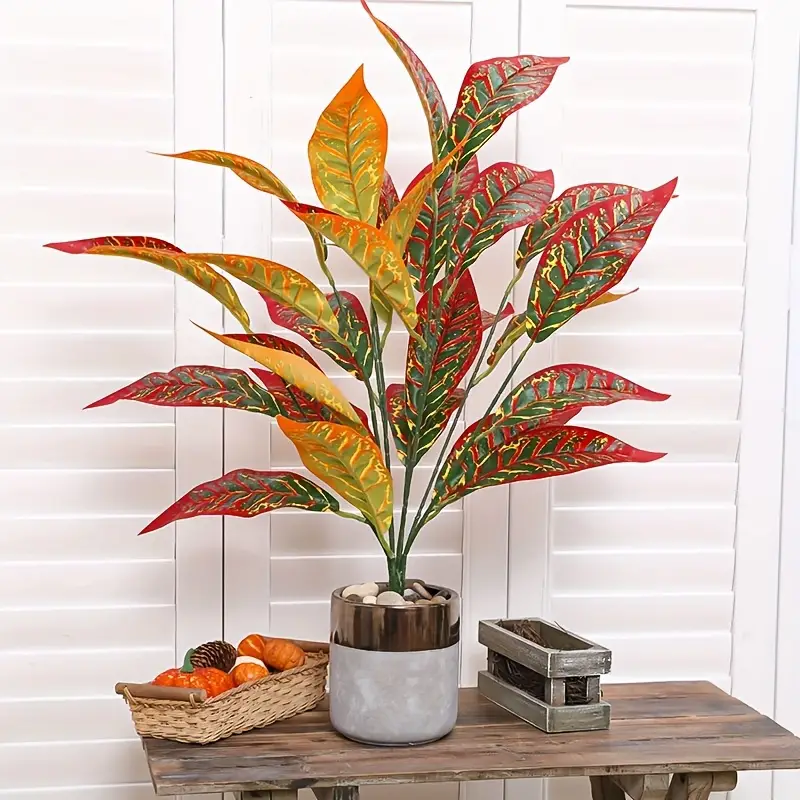This detailed color photograph showcases an indoor scene featuring a plant arrangement on a wooden table. The table, which has wooden legs, is placed in front of white wooden blinds that resemble bifold closet doors. The centerpiece of the scene is a tall, meticulously-kept plant, likely artificial due to its flawless appearance. The plant is housed in a stylish ceramic planter with a white base and a copper top, adorned with stones. The plant's branches have an array of colorful leaves, displaying shades of green, red, and yellow.

To the plant's left, there is a wooden box, possibly used for storage or decoration, containing elements like pine straw. To the right of the plant is a decorative basket filled with faux pumpkins and pine cones, adding an autumnal touch to the setting. The overall composition of the photograph suggests a curated and aesthetically pleasing indoor decor setup, blending natural elements with artificial enhancements.